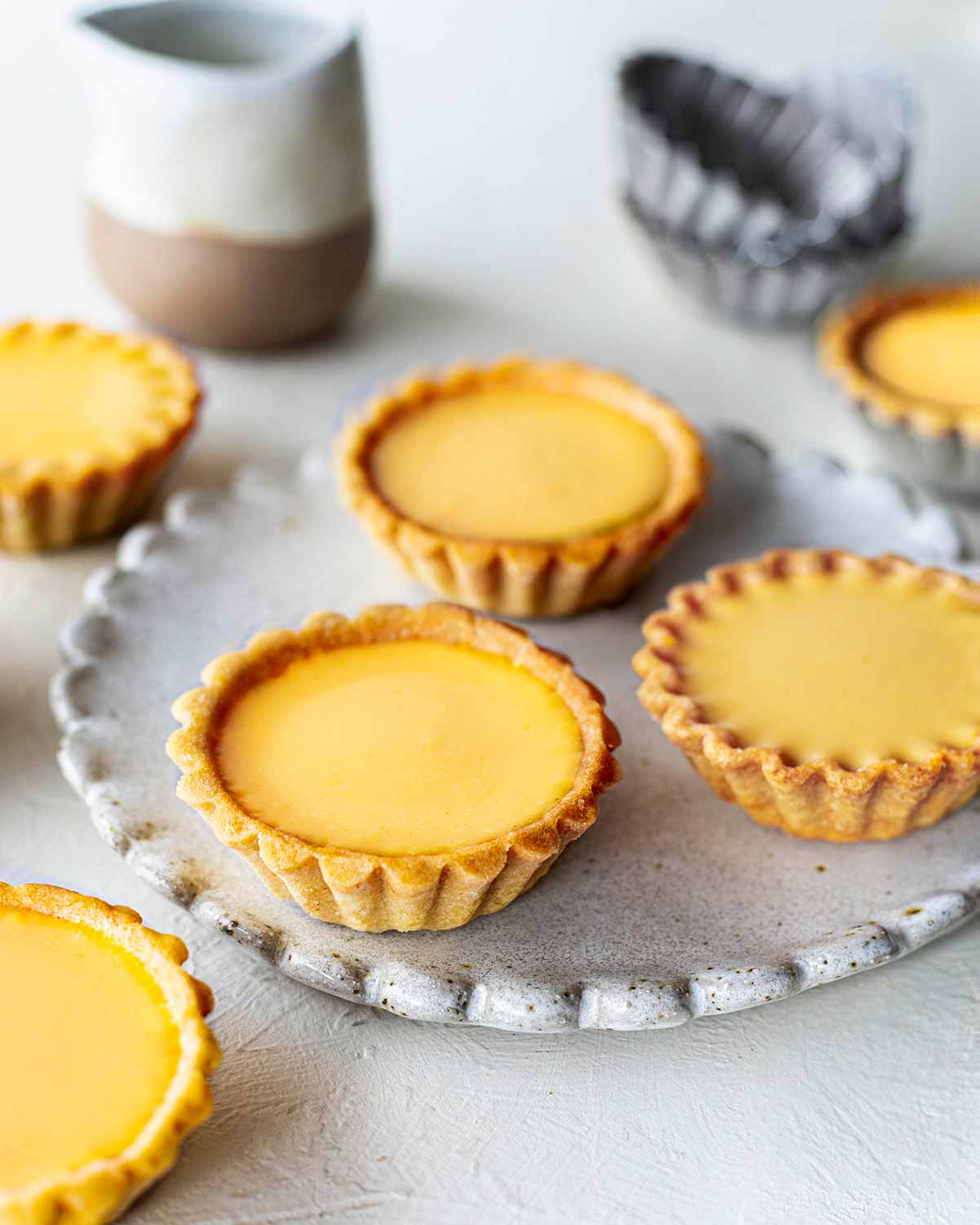This artistic photograph captures a serene and appetizing scene centered around delicate pastries. At the heart of the image on a textured white wooden table sits a gray plate with scalloped edges and subtle black accents, hinting at a weathered, rustic charm. The focal point is one of the three identical tarts with a vibrant yellow custard filling encased in a golden-brown crust. This tart, positioned towards the foreground, is sharply in focus, while the other two on the plate are gently blurred, forming a triangular arrangement. 

Behind the plate, additional elements contribute to the composition's depth: to the left, partially visible, is a tart alongside a piece of textured pottery; further along to the right, there is a stack of tart tins, partially obscuring another tart. In the top part of the image sits a stoneware pitcher, white at the top and brown at the base, adding an artisanal touch to the display. The overall color scheme of the photograph is predominantly white and neutral, which serves to highlight the vivid yellow of the custard, making the tarts the undeniable stars of this culinary still life.